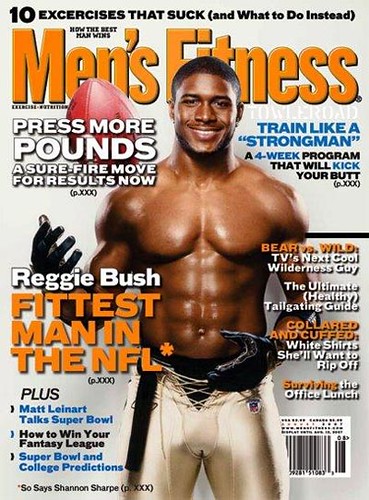The cover of Men's Fitness magazine features a bold, eye-catching design. The magazine title "Men's Fitness" is prominently displayed in bright orange letters. Above it, a headline in bold capitalization reads, "10 Exercises That Suck (And What To Do Instead)." The main focus of the cover is a highly muscular and toned African-American male, identified as Reggie Bush, who is a prominent NFL player. He stands at the center of the cover, facing forward, shirtless with his six-pack abs on display. He is dressed in tight, off-white, shiny football pants that are slightly undone at the top, revealing his black underwear. He wears black football gloves and is captured in mid-action, tossing an American football into the air.

Around the captivating image, several article titles are strategically placed. To the right of his head, a blue and black headline announces, "Train Like A Strongman: A 4-Week Program That Will Kick Your Butt." Below that, white and orange text highlights "Bear Vs Wild: TV's Next Cool Wilderness Guy," followed by "The Ultimate Healthy Tailgating Guide" in bold font. Under these, yellow letters spell out "Collared and Cuffed" and in white text, "White Shirt She'll Want To Rip Off," then in orange, "Surviving The Office Lunch." 

On the left side, near his chest, "Reggie Bush: Fittest Man in the NFL" is prominently displayed in white and orange text. Further down, additional features such as "Press More Pounds: A Sure Fire Move for Results Now" are in bold white letters with a black shadow. The cover also teases content on "Plus: Matt Leinart Talks Super Bowl," "How to Win Your Fantasy League," "Super Bowl and College Predictions," and "Shannon Sharpe," with a QR code at the bottom right corner for digital interaction.